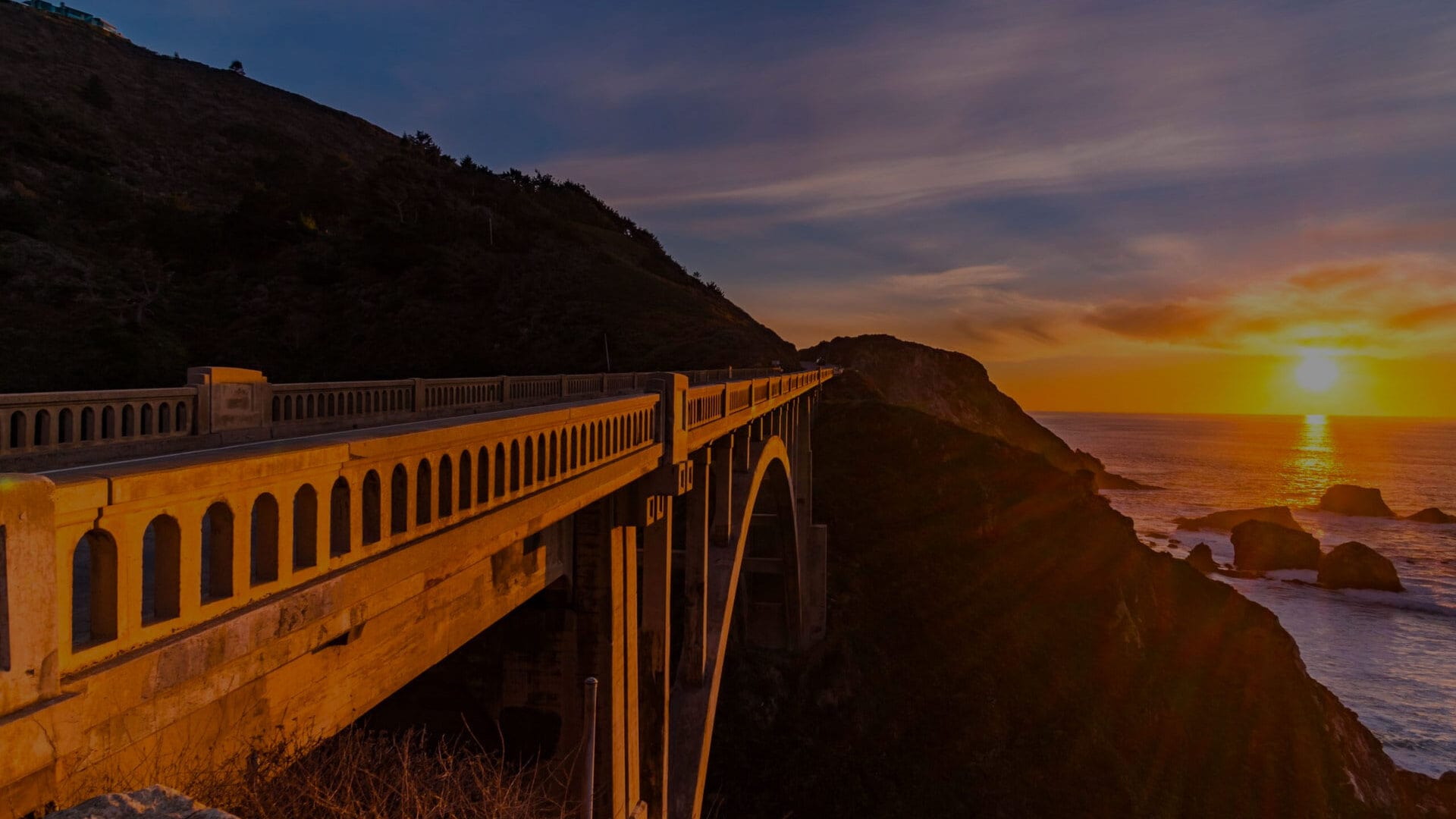This is a horizontal rectangular photograph taken at sunset, showcasing a large and long bridge that runs along the side of a high mountain. The bridge, though made of metal, appears almost wooden in the golden-brown glow cast by the setting sun. It features a railing and long stone pillars with arch formations underneath. The mountain beside the bridge is in shadow, with a darker hue and subtle goldish tint, revealing bits of outlined foliage.

To the right, the scene extends to an ocean sparkling under the sun's golden reflection. The water changes from orange at the horizon to a lighter whitish-blue closer to the viewer, peppered with big rocks. In the background, the sun is setting over the water, creating an orangey-yellow sky that gradually transitions to blue with streaks of purple and whispers of clouds. The overall view is a striking interplay of natural and man-made elements, captured from a vantage point that emphasizes the expanse and beauty of the landscape.